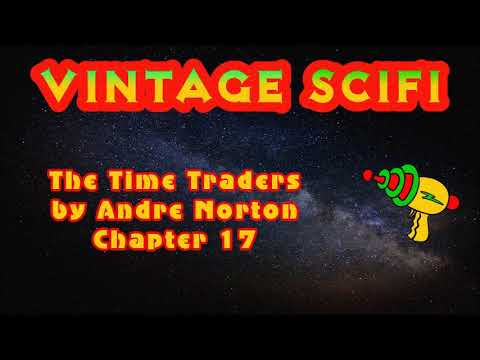The image is a vividly stylized title card with a night sky background featuring stars and nebulae moving diagonally from the upper left to the lower right. The top and bottom of the image are bordered by thick black bars. At the top, the large text "Vintage Sci-Fi" is prominently displayed in a bold font with a thick red outline and gradient letters transitioning from faded green to yellow. Below this, in smaller yellow text also outlined in red, are the words "The Time Traders by Andre Norton, Chapter 17," formatted onto three lines, aligned to the left. To the right of this text is a cartoonish depiction of a ray gun. This whimsical weapon has a yellow body adorned with a green "Z," a red dial at the back, and a muzzle featuring three progressively smaller green-rimmed, red-centered circles leading to a red cone tip ending in a red ball.